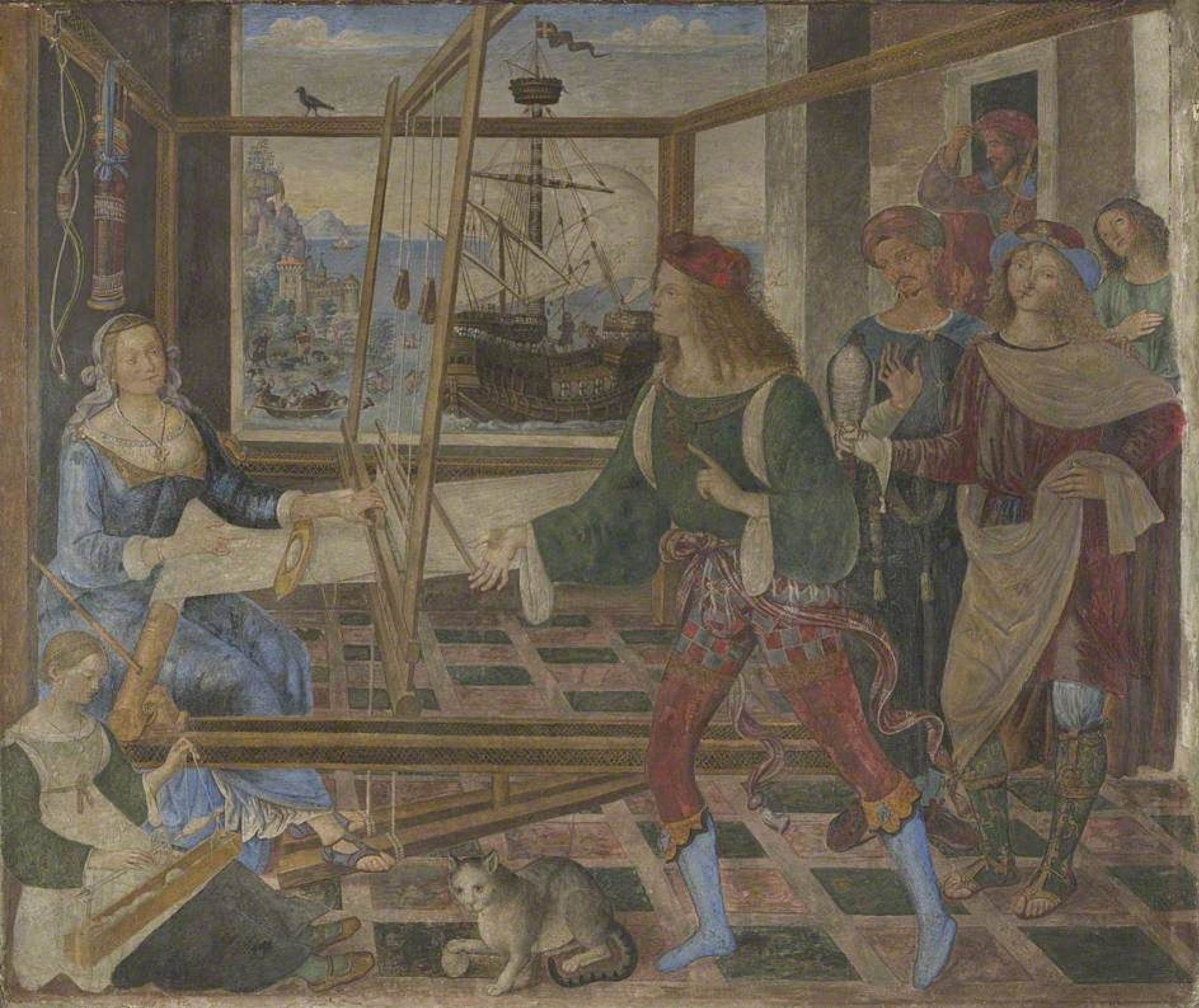The image, rendered in a detailed and colored pencil drawing reminiscent of Renaissance art, features a bustling indoor scene. On the left side, a woman in a blue dress is seated, seemingly weaving on a loom. At her feet, there is a younger woman, contributing to the busy atmosphere. The floor of the room is covered with square tiles and a gray cat is playfully pawing at something circular near its foot. On the right side of the image, four individuals, dressed in ancient-style robes and caps in blue, green, and red hues, are entering through a doorway. One of these figures, a man with shoulder-length hair, appears to be speaking to the woman by the loom. In the background, a window looks out onto a sea scene with a majestic brown ship sailing on blue waters, further complemented by glimpses of a castle. The image has a dark and grainy quality, lending a faded and historical European aesthetic to the vibrant activity inside the hall.